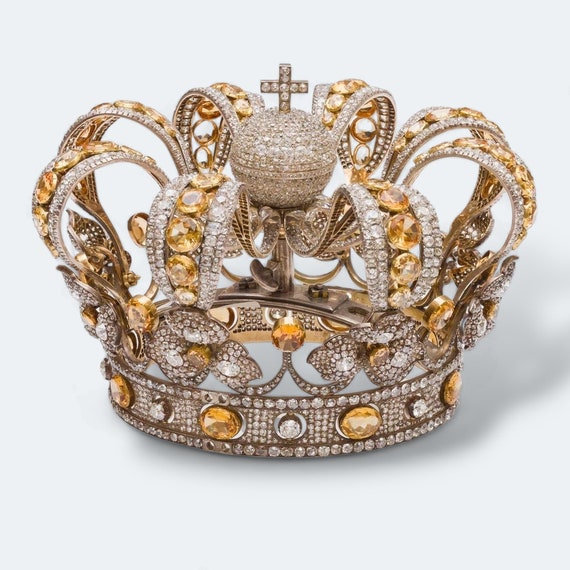This image showcases a highly ornate and holy crown, adorned with an array of sparkling jewels. The crown features numerous diamonds and yellow gemstones, which appear to be yellow topaz or golden yellow diamonds, surrounding its intricate structure. A band of small diamonds encircles the base, followed by rows of larger diamonds interspersed with substantial yellow gemstones meticulously placed around the circumference. At the crown's pinnacle, a diamond-encrusted sphere is topped with a prominent cross, emphasizing its religious significance. The gems are arranged in various shapes, adding to the crown's dazzling and regal appearance. The detailed craftsmanship and the distribution of diamonds and yellow gems, potentially forming floral or fleur-de-lis patterns, contribute to its elaborate and majestic design, suggesting it may belong to a notable religious or royal collection, possibly British or French.